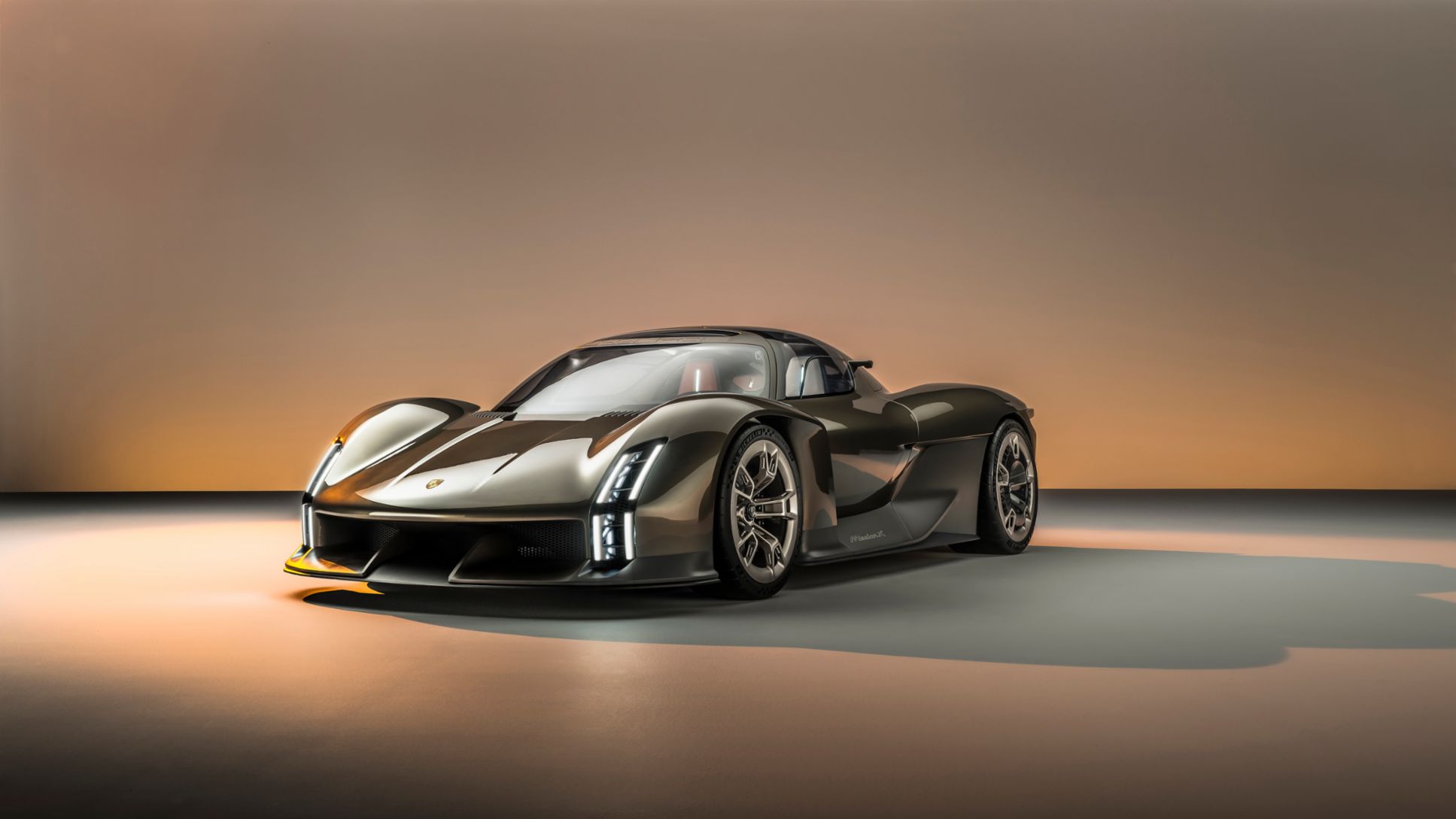The photograph features a sleek, dark gray sports car centrally located in a horizontal rectangular frame that is wider than it is tall. The car, which appears to be a prototype or a collector's model, is showcased in a monochromatic interior space with a golden-gray hue. Soft, bright lighting from the left side of the frame accentuates the car's incredibly shiny, sculpted metal surface, casting dramatic shadows on the smooth, reflective floor. The image captures the car in a three-quarter profile, facing the left towards the camera, highlighting its aerodynamic yet slightly unusual design. Notably, the headlights are long, vertical rectangles, adding to the modern, new-age aesthetic. The car’s wheels sport higher arches compared to the low front hood, enhancing its futuristic look. The creamy pinkish-gray background complements the metallic sheen of the car, and the car's shadow is prominent on the right side, adding depth to the scene.